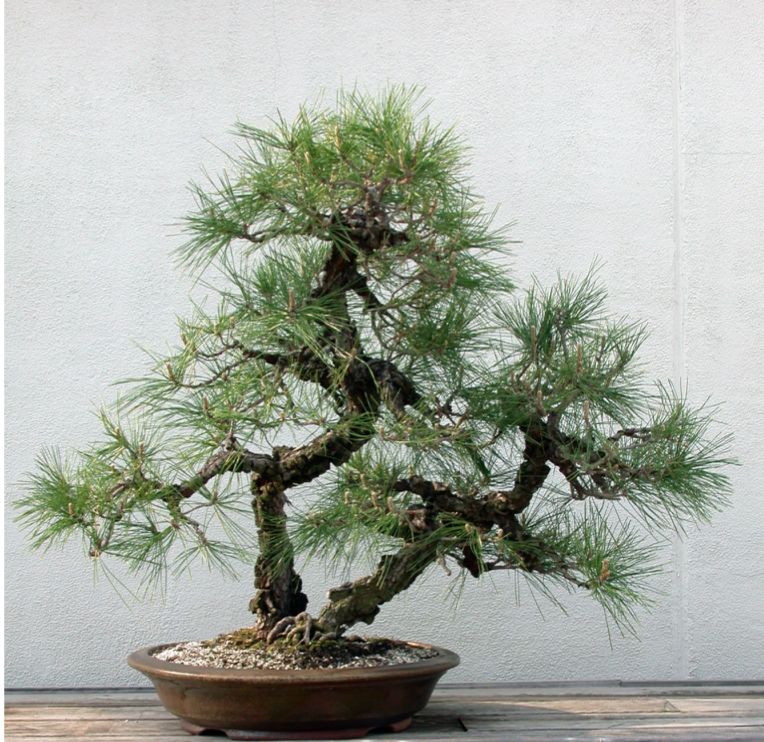This detailed photograph features a black pine bonsai tree displayed in a narrow but wide circular dish adorned with pebbles. The bonsai consists of two distinct parts that grow together, each resembling small, individual trees. The right tree trunk extends outward and leans to the right, showcasing its shaggy brown bark. Both parts exhibit green, prickly pine needles at the ends of their branches.

The bonsai is prominently positioned in the center of the image, which appears to be taken indoors, potentially within someone's home. The tree sits on a wooden surface, which is brown and aligns with a visually similar brown counter or table. The backdrop showcases a stucco white wall, adding a textured and contrasting background to the scene, enhancing the focus on the intricate details of the bonsai tree.